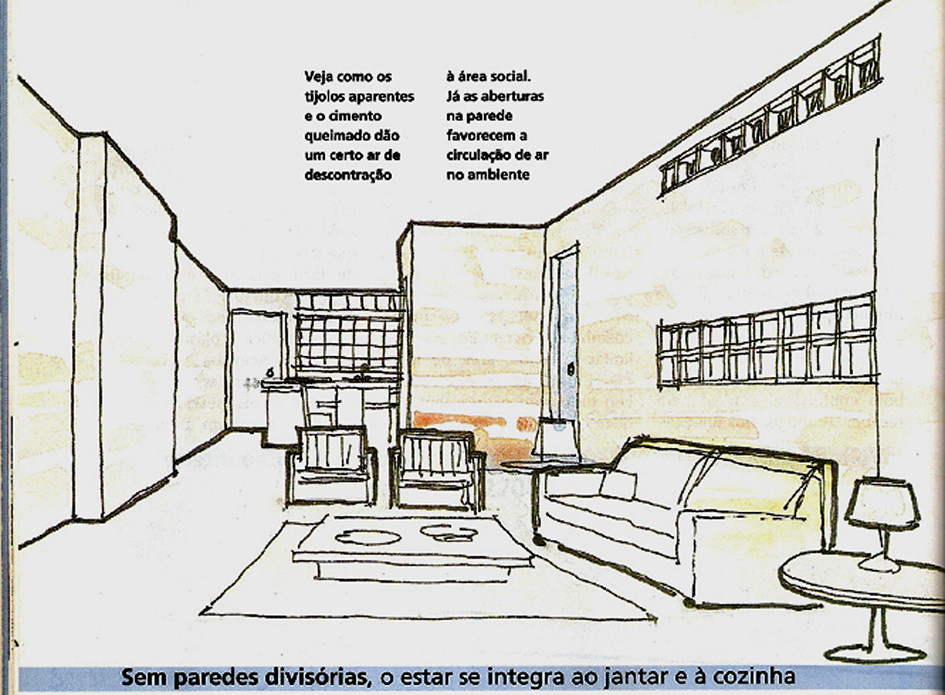This image is a detailed hand-drawn rendering of a living room captured on a piece of paper, possibly taken out of a book. The primary medium appears to be pen or black ink. The living room is an open concept space that connects to a kitchen in the background, which features a kitchen counter and distinctive tiles on the wall. Central to the living room, a sofa is placed against the wall beneath a series of large glass windows, with one prominent picture window below a long, narrow transom window. In front of the sofa, a coffee table rests on a rug, flanked by two chairs. To the bottom right, a round end table with a lamp adds detail to the scene. The walls are colored in shades of brown, gray, light pale yellow, and orange, evoking a sandy palette. There is text on the page which is not in English, describing the visual contrast of the tiles and the cement, and noting the openings in the wall that aid in air circulation throughout the space.